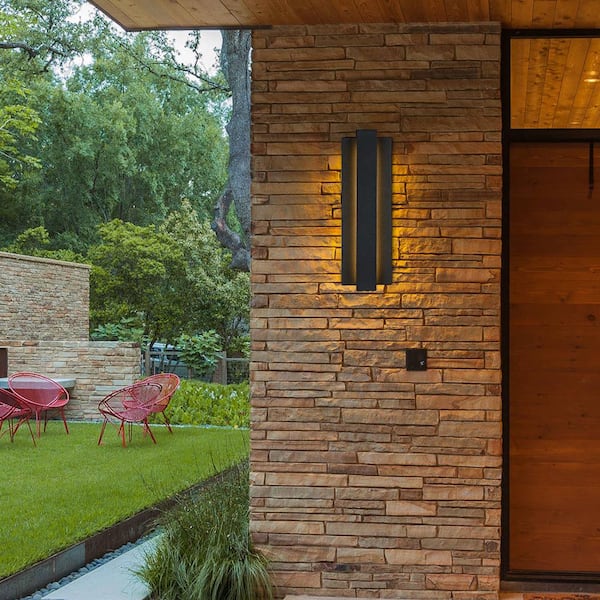This image portrays the exterior of a home and its adjacent backyard, merging elements of all three descriptions for a detailed view. The entryway is located on the right side, marked by a dark brown wooden door with a small glass window above it. Adjacent to the door is a pillar constructed from thin, reddish-brown sandstone bricks laid one on top of the other, contributing to the home's rustic aesthetic. Mounted on this pillar is a rectangular, black light fixture, emitting a soft yellow glow, beside which is a black buzzer.

To the left of the entryway extends a short stone wall, composed of brown sandstone blocks. Adjacent to the wall, a gray sidewalk leads to a lush, emerald-green lawn in the backyard. The yard features four circular, basket-like, red patio chairs, perfectly arranged on the freshly mown grass, offering a vibrant seating area. Behind the chairs, a robust stone wall stretches across the yard, providing a sense of enclosure.

Beyond the wall, a variety of tall trees, their dense green foliage reaching up towards a partly cloudy sky, form a picturesque backdrop. These trees have broad gray trunks and are bathed in a gentle glow of sunlight filtering through the leaves. Overall, the scene captures a harmonious blend of natural and architectural elements, creating a serene and inviting outdoor space.